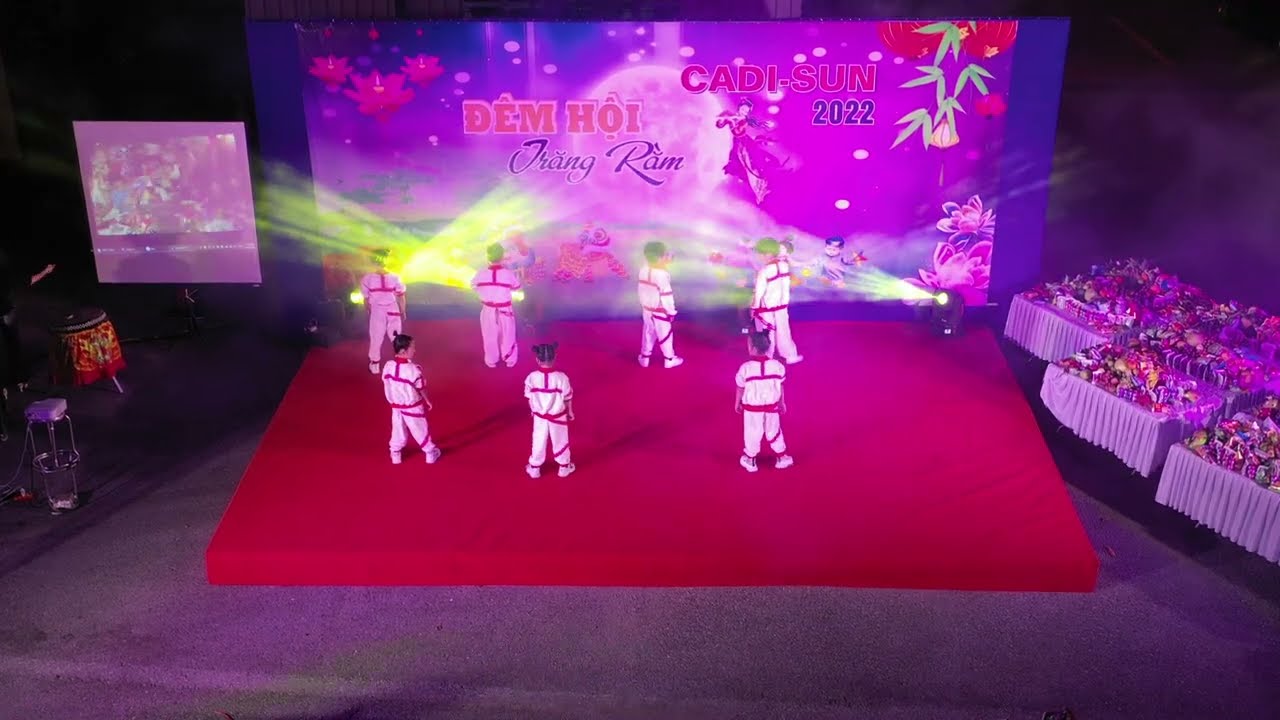In this detailed landscape-oriented color photograph taken from above, we see seven young children standing on a red platform that is positioned on a purple carpeted surface. The children, who appear to be part of a dance troupe or performance group, are dressed in white jumpsuits with red trim and have their backs turned to the camera. Three children are closest to the camera, and four are further away.

In the background, there is a large screen with text in Vietnamese that reads "Dem Hoi Trang Ram" and "KADI-sun 2022." This screen is part of a mural with an Asian motif featuring flowers, leaves, a white ball at the center, and beams of light. To the left of the main screen, there is a smaller, less discernible screen.

On the right side of the purple carpeted area, there are tables covered with white pleated tablecloths, set up with various objects that appear to be gifts or possibly food. Additionally, stools are scattered on the purple carpeted surface. The photograph is lit by spotlights placed at the corners of the stage, enhancing the vibrant colors and details of the scene.